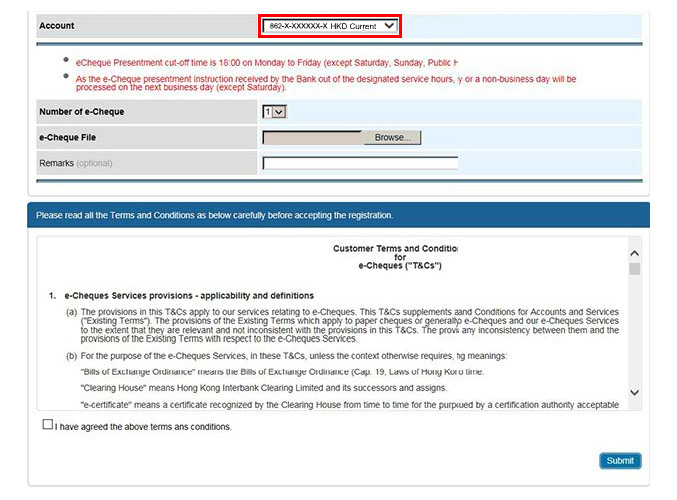The image displays a user interface with multiple elements related to financial account management. 

At the top, there is a label titled "Account". Below it, a red box highlights a text entry field displaying "862-X-XXX" followed by some letters and the word "current." This suggests that certain digits are masked or restricted from further disclosure.

Next to this, there is a dropdown arrow. Adjacent to it, there’s text stating "E-Check present cut off time is 1800 on Monday through Friday except Saturday Sunday public," which seems to be cut off and incomplete. It is likely informing users about the cutoff times for E-Check transactions within the specified days excluding weekends and public holidays.

There is an unclear section questioning "Is E-Check presentment instruction received by the bank of the designated service hours?" suggesting possible typos or confusing phrasing.

Below, a field shows the "Number of E-Checks" as filled in with the number one.

Further down, there’s a section titled "Customer Terms and Conditions," but the text implies incomplete or missing information, leading to a suspicion regarding the site's trustworthiness.

Lastly, there is an option to click on "I’ve read the above terms," indicating user confirmation of understanding the terms displayed.